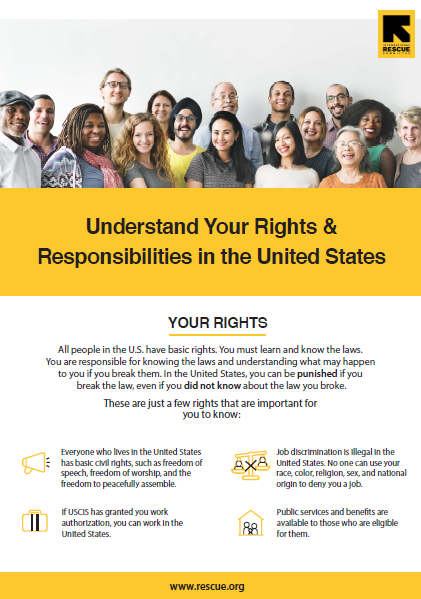The image features an informational support page designed to educate individuals about their rights and responsibilities in the United States. At the top of the page is a photograph depicting a group of people, possibly representing a foundation or organization dedicated to supporting community members. Below the photograph, a prominent yellow rectangle contains the text: "Understand Your Rights and Responsibilities in the United States."

The text emphasizes that all individuals in the U.S. possess basic rights and underscores the importance of learning and adhering to the law. It highlights that ignorance of the law is not an excuse and that legal consequences will follow if laws are broken.

Key points mentioned in the text include:
- The importance of knowing the laws and the implications of breaking them.
- Fundamental civil rights enjoyed by everyone in the U.S., such as freedom of speech, freedom of worship, and the right to peacefully assemble.
- Employment rights, clarifying that work authorization from USCIS permits individuals to work, and emphasizing that job discrimination based on race, color, religion, sex, or national origin is illegal.
- Availability of public services and benefits for eligible individuals.

At the bottom of the page, the website address www.rescue.org is listed, indicating a potential resource for further information and support.